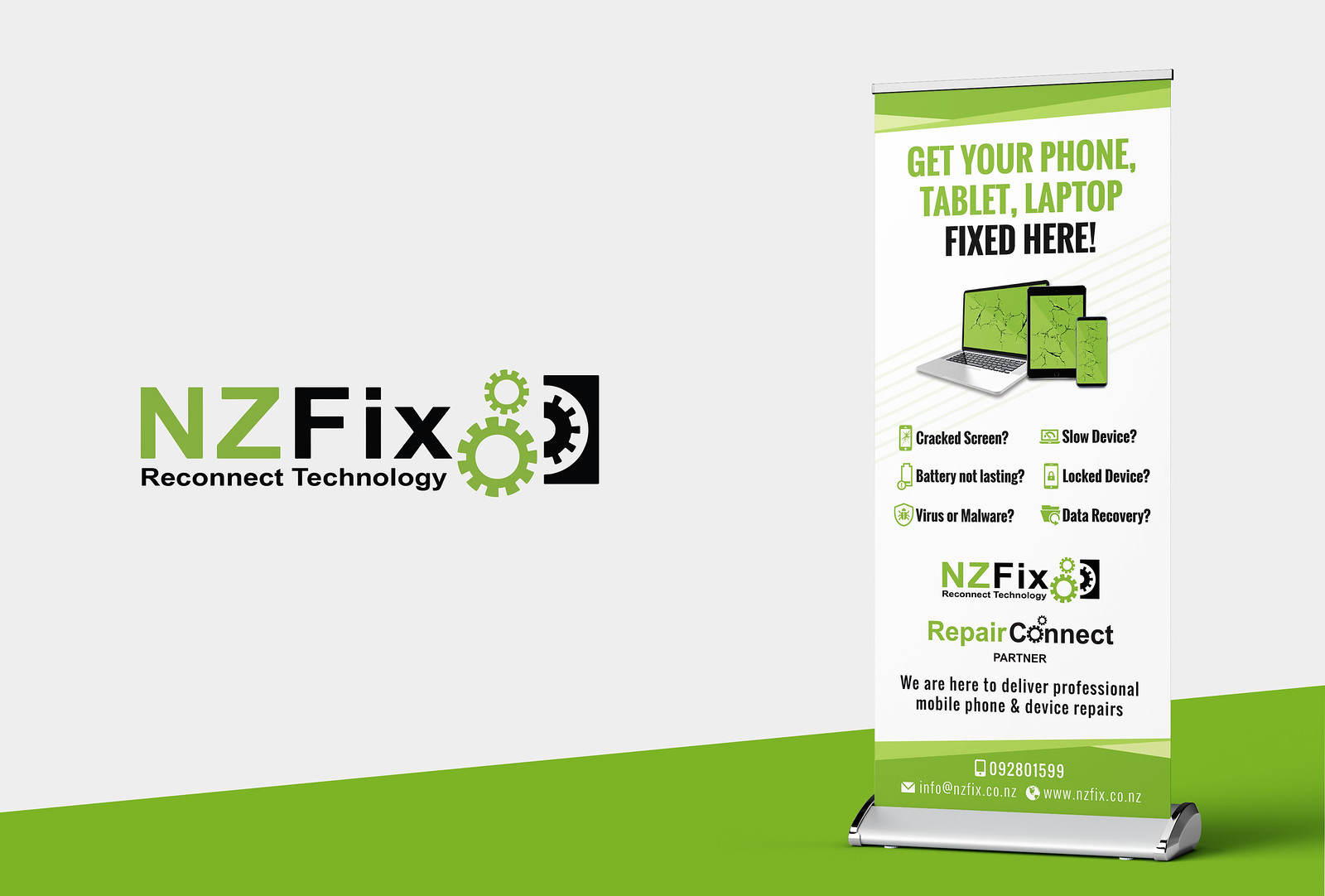The promotional flyer for NZFix Reconnect Technology features a predominantly light gray background with a striking green triangular section extending from the bottom left corner to slightly above the bottom right corner. On the left side of the image, the bold black letters "NZ Fix" are prominently displayed, accompanied by green and black gears, with the accompanying phrase "Reconnect Technology" below. 

To the right of the logo, a pop-up promotional banner mirrors the flyer’s gray and green color scheme, with green borders at the top and bottom. The banner prominently reads "Get Your Phone, Tablet, Laptop Fixed Here" in green and black font. Below this, there's a detailed illustration showing a laptop, a tablet, and a cell phone, each depicting common repair issues such as cracked screens, battery problems, slow performance, viruses or malware, locked devices, and data recovery. The banner also reiterates the logo and highlights their repair services, identifying them as a Repair Connect Partner, committed to delivering professional mobile phone and device repairs. Contact information including the phone number, email, and website is listed at the bottom of the banner.